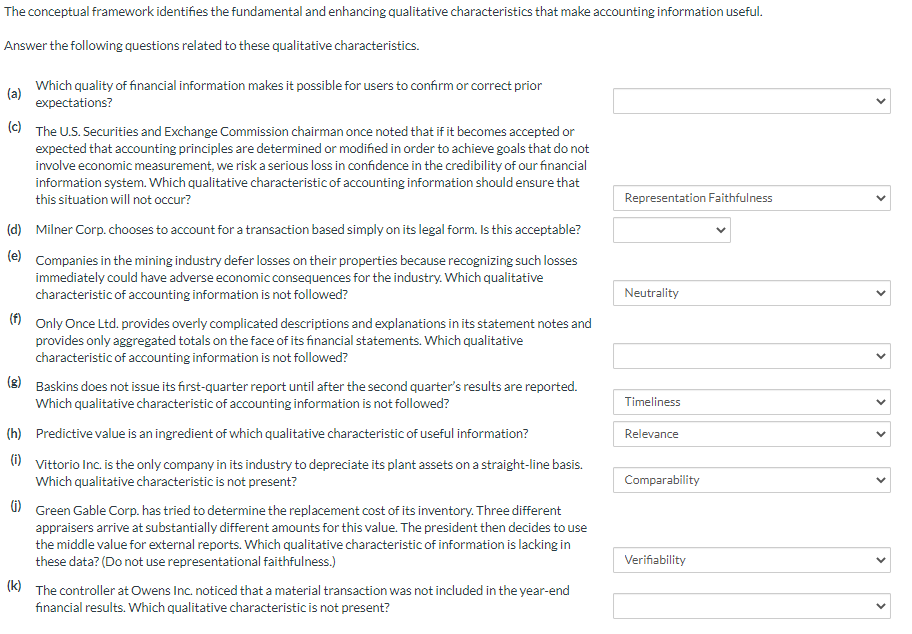**Detailed Caption:**

On a clean white background, the text outlines a conceptual framework that delineates the essential and enhancing qualitative characteristics that render accounting information useful. The text presents a series of questions aimed at exploring these qualitative characteristics in depth:

1. **Question A:** Which quality of financial information enables users to confirm or correct prior expectations?
2. **Question C:** The U.S. Security and Exchange Commission chairman once noted that if it becomes accepted or anticipated that accounting principles are established or altered to achieve aims that do not involve economic measurement, there is a significant risk of losing confidence in the credibility of our financial information system. Which qualitative characteristic of accounting information should prevent this from happening?
3. **Question D:** Is it acceptable for Milner Corporation to choose to account for a transaction solely based on its legal form?
4. **Question E:** Companies within the mining industry often defer losses on their properties because immediate recognition of such losses could have detrimental economic impacts on the industry. Which qualitative characteristic of accounting information is not being adhered to in this scenario?

The framework and questions seek to highlight the importance of adhering to qualitative characteristics to ensure the reliability, comparability, and transparency of financial information.